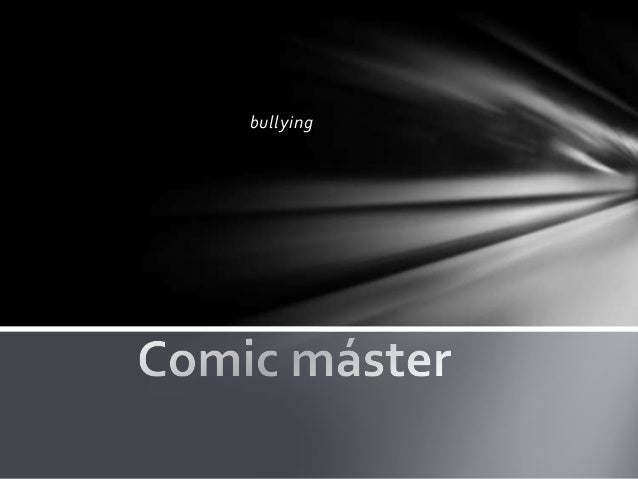The image is divided into two unequal sections by a white line, forming a box frame. The top section, which takes up roughly two-thirds of the image, features a black background with white rays emanating from the top right corner, creating a mirage-like effect across the section. In the middle of this section, the word "bullying" is written in small, italicized, lowercase white letters. The bottom section is about a third of the image size and has a gradient background transitioning from darker gray on the left to lighter gray on the right. This section contains the text "Comic Master" in a larger font compared to "bullying," with the letter "A" in "Master" accented. The composition contrasts the dark, dramatic top half with a calmer, gradient bottom half, using text size and background colors to convey a nuanced visual message.